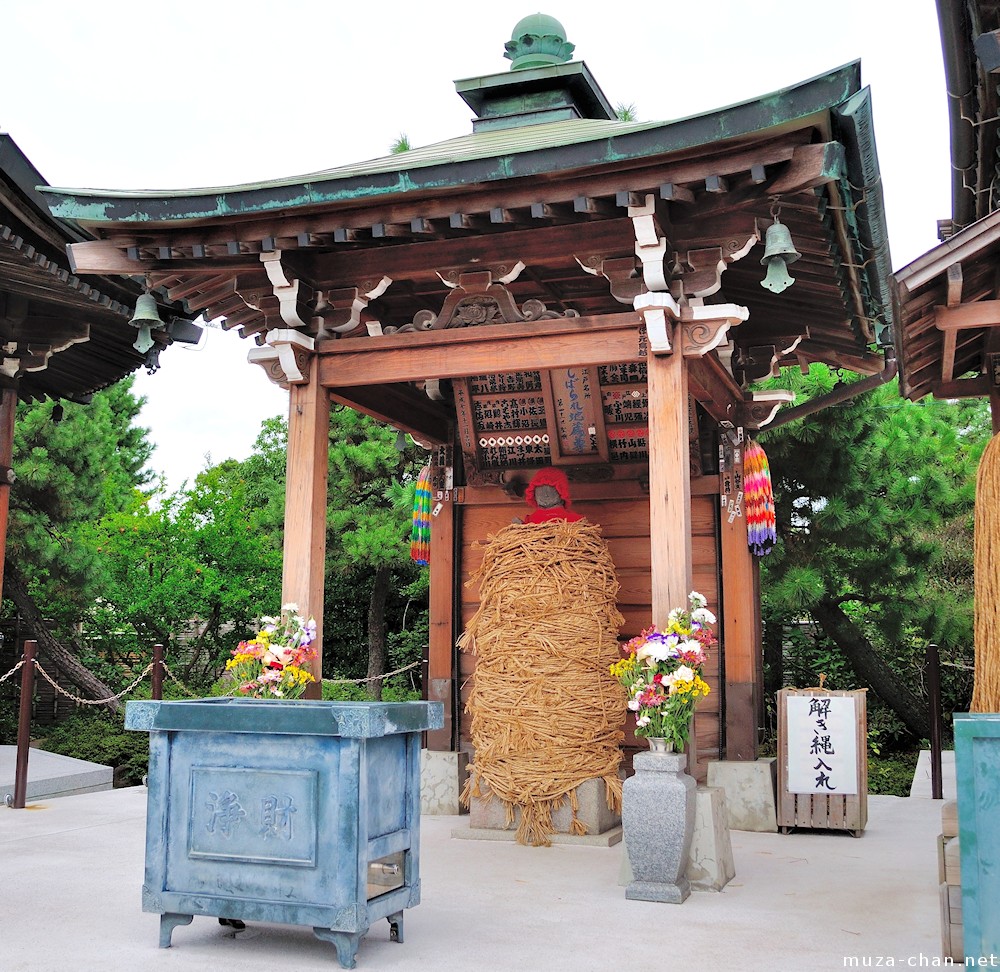This color photograph captures a serene outdoor scene in Japan featuring a traditional Japanese shrine. The image, oriented in a square format, is meticulously detailed: the backdrop showcases a nearly white sky, hinting at light blue, with a lush line of vivid green trees. Dominating the scene is a classic Japanese-style pavilion, characterized by a roof that curves gracefully at each corner, ascending to a central flat section topped with a rounded, greenish-blue ornament that resembles patinated copper. 

The roof is supported by vertical wooden struts and robust horizontal beams. Beneath this intricate wooden structure resides a striking effigy adorned with a red hat and a matching red top, enveloped in what appears to be a bale of fluffy hay or straw. This figure seemingly rests on a platform that may serve religious or commemorative purposes.

Surrounding the effigy are various stone flower holders, each filled with vibrant, colorful flowers. To the left in the foreground, a blue stone-like box or altar with flowers placed on it forms part of the scene. Additional elements include walkway poles connected by rope-style chains that guide visitors, and hanging multi-colored ornaments or windsocks. The scene's cleanliness adds to its solemn, reflective atmosphere. A textual marking "MUZA-CHAM.net" is imprinted in the bottom right corner of the photograph.